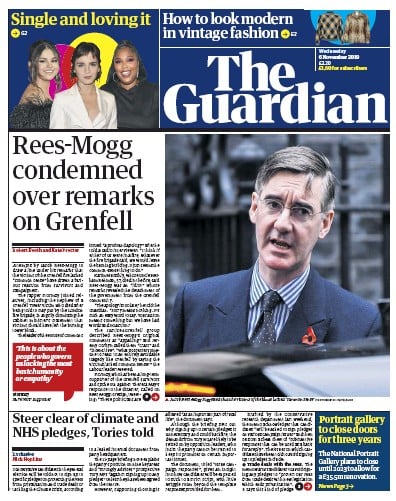The cover of The Guardian magazine features a visually engaging collage of text and images. In the top left corner, bold yellow text declares, "Single and Loving It," accompanied by images of entertainers such as Lizzo and Selena Gomez. To the right, under the heading "How to Look Modern in Vintage Fashion," a stylish black and yellow sweater is displayed next to a chic brown jacket.

Centered prominently on the cover is a photograph of a man with a slightly open mouth, black eyebrows, and black hair streaked with gray, giving off an air of stress or irritation. He dons a blue and white striped collared shirt, a navy blue suit jacket, and a matching tie. To the immediate left of his image, white text reads, "Rees-Mogg Condemned Over Remarks on Grenfell."

In the bottom left section, more headlines draw attention, including "Steer Clear of Climate and NHS Pledges, Torres Told." Finally, on the right side, enclosed in a navy blue rectangle, the caption "Portrait Gallery to Close Doors for Three Years" announces a significant cultural update.

The impeccable arrangement of text and imagery encapsulates the dynamic range of stories covered by The Guardian, engaging readers with its visually compelling and informative presentation.